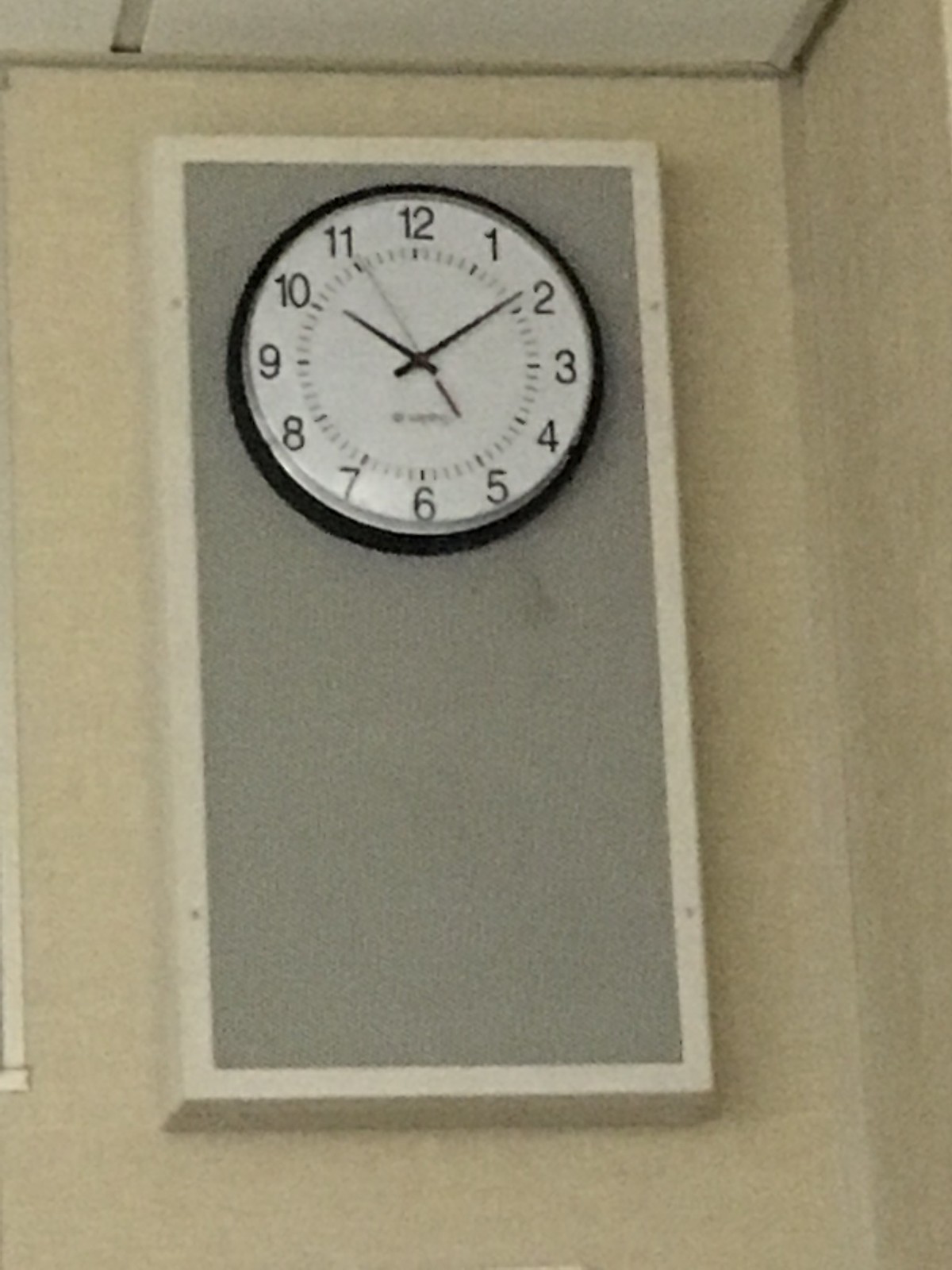The image showcases a wall with a gray or beige background. In the center, a white rectangular recess houses a clock. The clock itself features a black rim and a white face with black numerals and hands. Although there is a brand name imprinted on the lower half of the clock face, it is too blurry to discern clearly. The time displayed on the clock is approximately 10:09. Above the clock, the ceiling is composed of tiled panels.